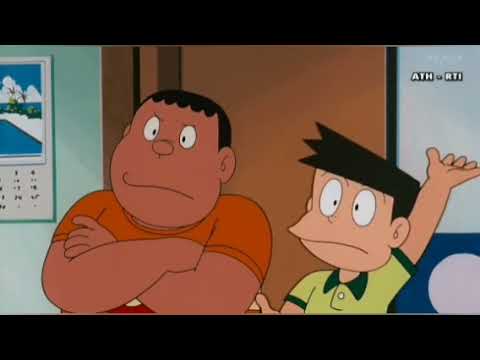In this cartoon image, set in what seems to be a classroom, two school boys stand in front of a light bluish-gray wall with a brown door centrally located behind them. A portion of a calendar is visible on the left side of the wall. The larger boy on the left has brown skin and short, dark curly hair. He has big white oval eyes with black pupils and a circular nose. Dressed in an orange t-shirt, he appears frustrated or angry, with his arms crossed and a curved line on his face indicating his displeasure. The smaller boy on the right, who is light-skinned, features straight, pointy hair and a long, curved line for a mouth. He has equally large oval eyes and a pointy nose. Wearing a light green shirt with a dark green collar, he raises his left hand excitedly, perhaps signaling eagerness or the act of asking a question. The top right of the frame shows the text "A-T-H - R-T-I," suggesting a low-resolution capture from a video.